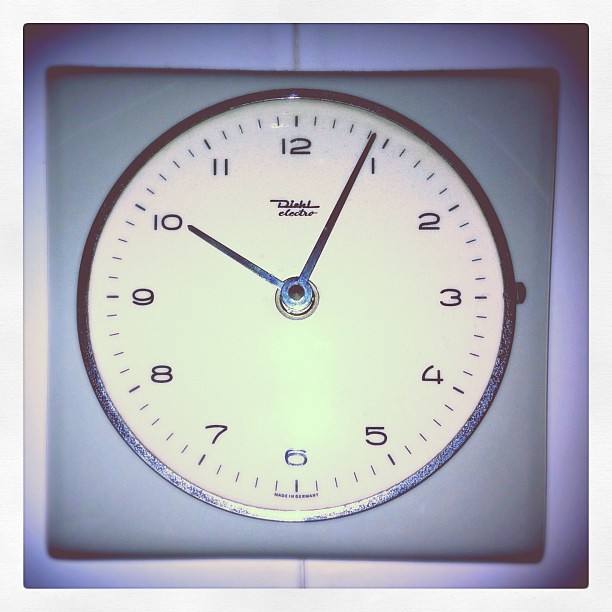This photograph features an antique or vintage-style clock, characterized by its retro font and old-fashioned design. The clock face is circular with a white background and black numbers, encased in a large, square green frame. The black metal hour and minute hands point to approximately 10:04. Notably, the clock lacks a second hand and has a thin, distinctive font for its numbers. Above the 12, the name "Diablo Electric" is inscribed, and at the bottom, it reads "Made in Germany." The clock is mounted on a tiled, purple wall, which may be a counter or table, and the photograph includes a thick white border around the image, highlighting the clock's unique design.